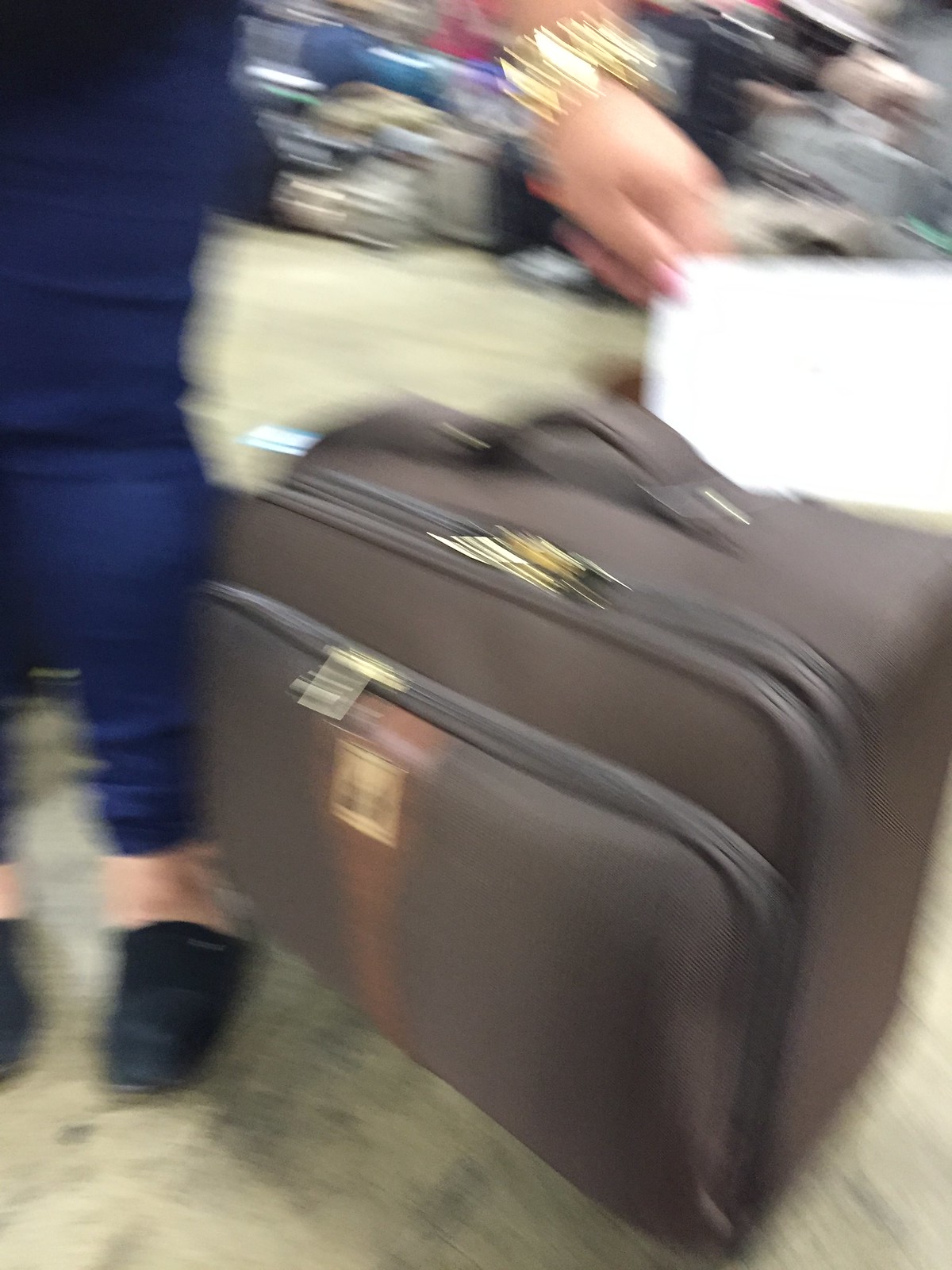In this very blurry image, a person stands next to a large, brown, full-size suitcase, likely suited for air travel or long trips, with solid sides, two zippered compartments, and a prominent brown handle. The individual is dressed in brown pants and dark-colored, possibly black, slip-on shoes, with their light-colored skin visible around the feet. They are wearing gold jewelry on their wrist, although the details are obscured due to the blur. The person holds a flat, white sheet of paper or a similar object in their light-skinned hand, without any visible writing discernible. The backdrop is equally blurred, with what appears to be a stack of additional luggage. The scene is set on a light beige ground.